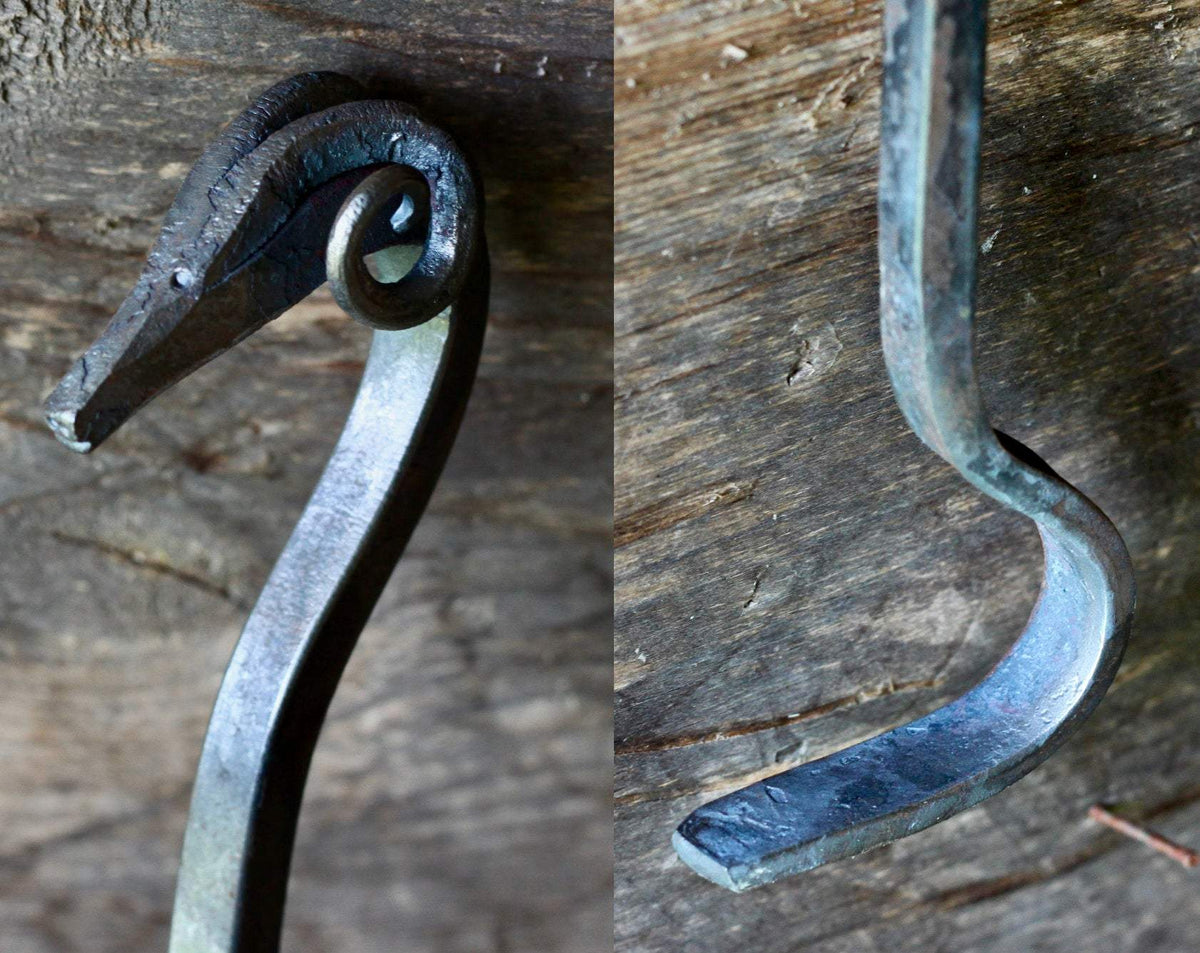The image features two color photographs, presented side-by-side in a landscape orientation. Each photograph showcases a different view of a rod iron tool, set against a dark gray, weathered barnwood surface, possibly an old wooden table or floor. 

On the left side, the tool, which is dark metal with hints of green and rust from oxidation, has a square rod that curves at the top. The texture of the metal changes as it becomes rough and ends in a point with an additional twist, resembling the curled horns of a mountain goat. Below this head-like feature, the rod transitions into a handle-shaped flat piece of metal.

On the right side, the same tool is viewed from the opposite end. Here, the curving part of the rod is positioned at the bottom, flattening out towards the handle. Throughout, the realistic, representational photographic style highlights the tool's intricate details, underscoring its handcrafted appearance and functional design as a potential fireplace or log-pulling tool.